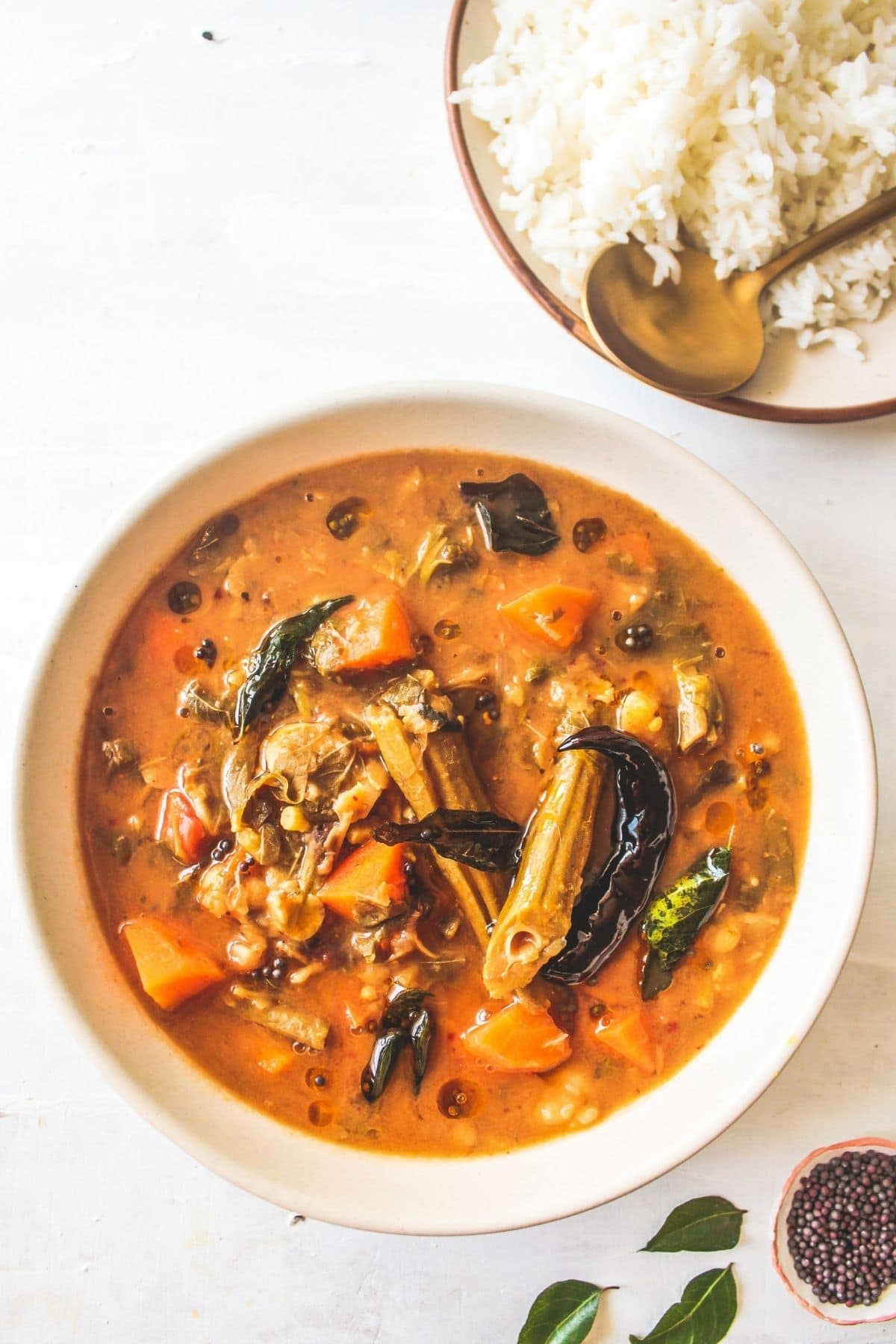An aerial photo captures an off-white kitchen table setting showcasing two distinct bowls of food. In the foreground, a white bowl with a creamy soup takes center stage, its vibrant orange broth adorned with chunks of vegetable or meat, including hues of black, yellow, and orange—possibly pieces of carrot and other ingredients. Floating atop the soup, there are also a few green leaves, suggesting aromatic herbs. To the top right, a second bowl, characterized by its white body and brown rim, contains a serving of white rice, accompanied by a gold spoon resting inside. Decorating the bottom right corner of the image, three green bay leaves are carefully arranged next to a small cluster of red, white, and black peppercorns, adding a touch of culinary spice to the composition. The overall backdrop is a light gray, slightly shaded on the right, highlighting the minimalistic and tasteful arrangement of this appetizing scene.